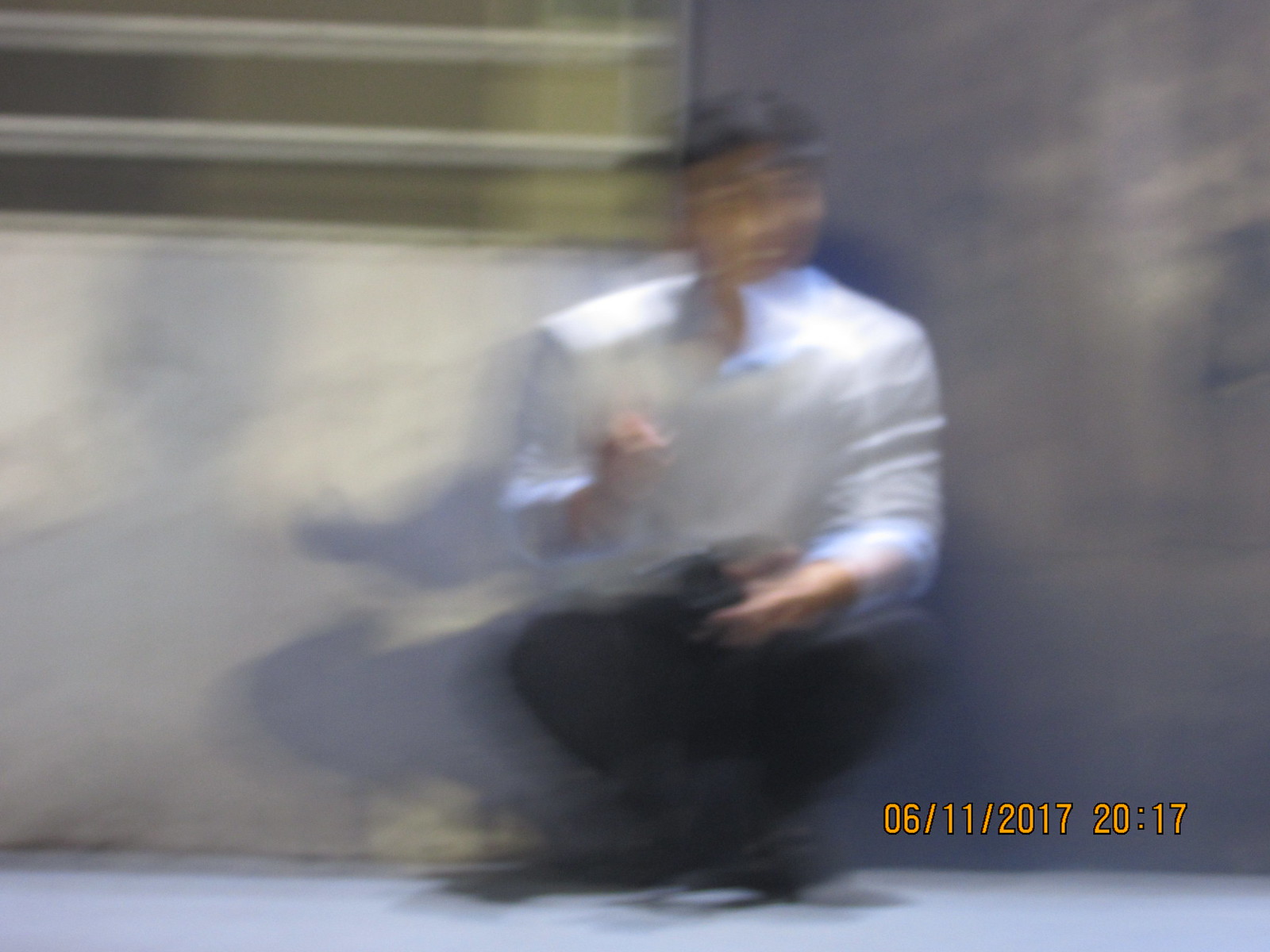In this blurred photograph dated June 11, 2017 at 8:17 PM, we see an Asian man squatting down on what might be a sidewalk or at a bus station. The background features a mix of white and dark gray walls, with the left side presenting a textured white concrete wall adorned with horizontal railings, and a hint of yellow peeking above. The right wall transitions from a light center to a darker gray hue. The man, with dark hair, is dressed in a white collared shirt resembling a chef's jacket and black pants. He is squatting with his ankles crossed, his right hand bent at the elbow near his chest, while his left hand rests on his thigh, holding a black object. The overall image is quite blurry, possibly due to motion or deliberate editing. A date stamp on the bottom right corner confirms the timestamp.